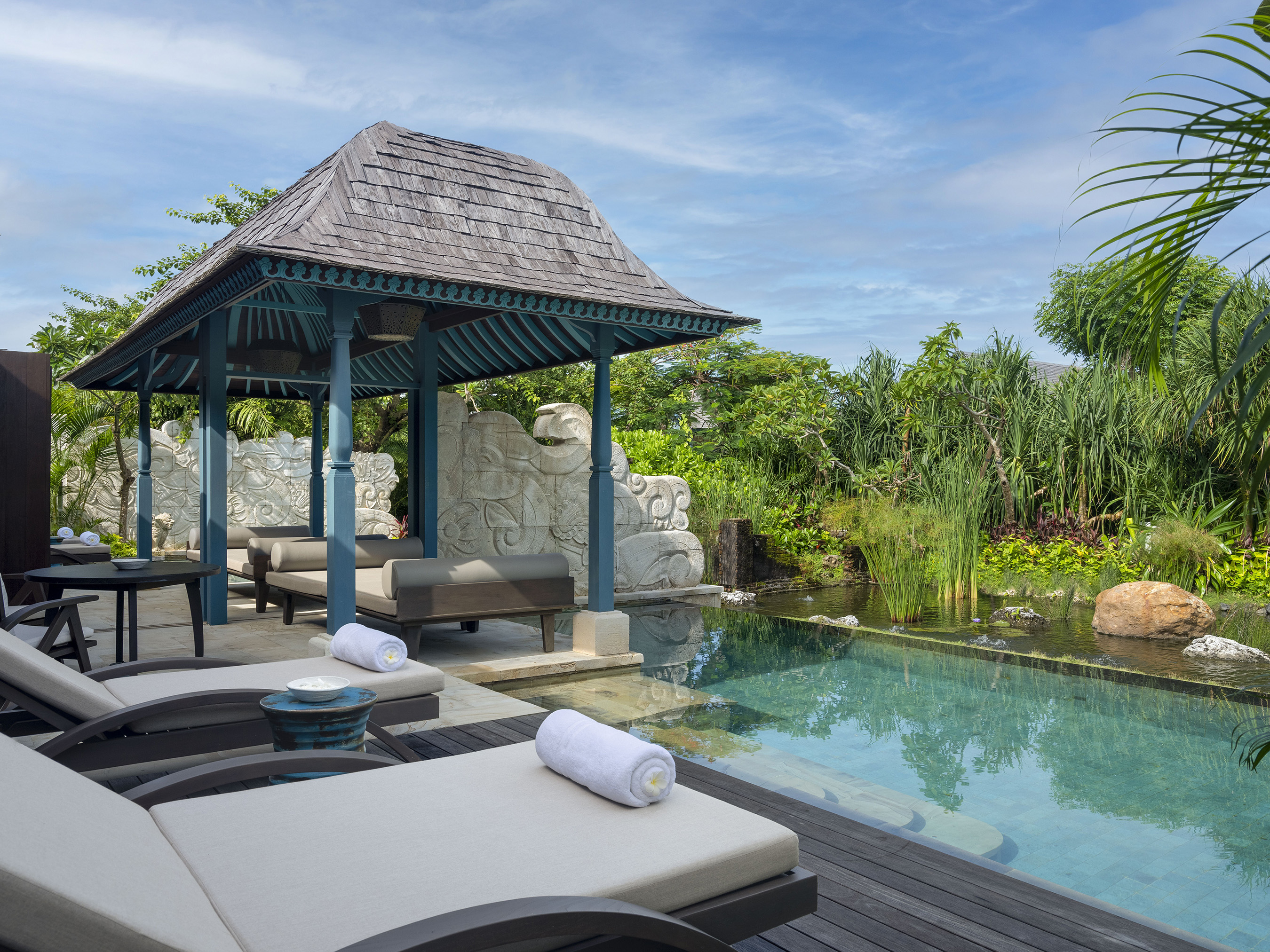The photograph captures a serene tropical backyard setting under a soft blue sky dotted with white, scattered clouds. Dominating the scene is a modestly-sized but inviting rectangular swimming pool with a surrounding gray wooden patio. To the left of the pool, a set of comfortable white beach chairs with gray bases and neatly rolled white towels provide an inviting spot for relaxation. The vibrant greenery of low-growing tropical trees and fronds encircles the area, offering a lush and controlled natural backdrop.

In the background, a gentle hill enhances the tropical ambiance. A pavilion with a shingled roof and green interior paint stands prominently, complete with green support beams. Underneath this canopy, two large, cushioned outdoor beds, each adorned with rolled pillows, offer luxurious lounging spaces. The overall composition of the image exudes tranquility and leisure, encapsulated within a picturesque and well-maintained tropical garden.